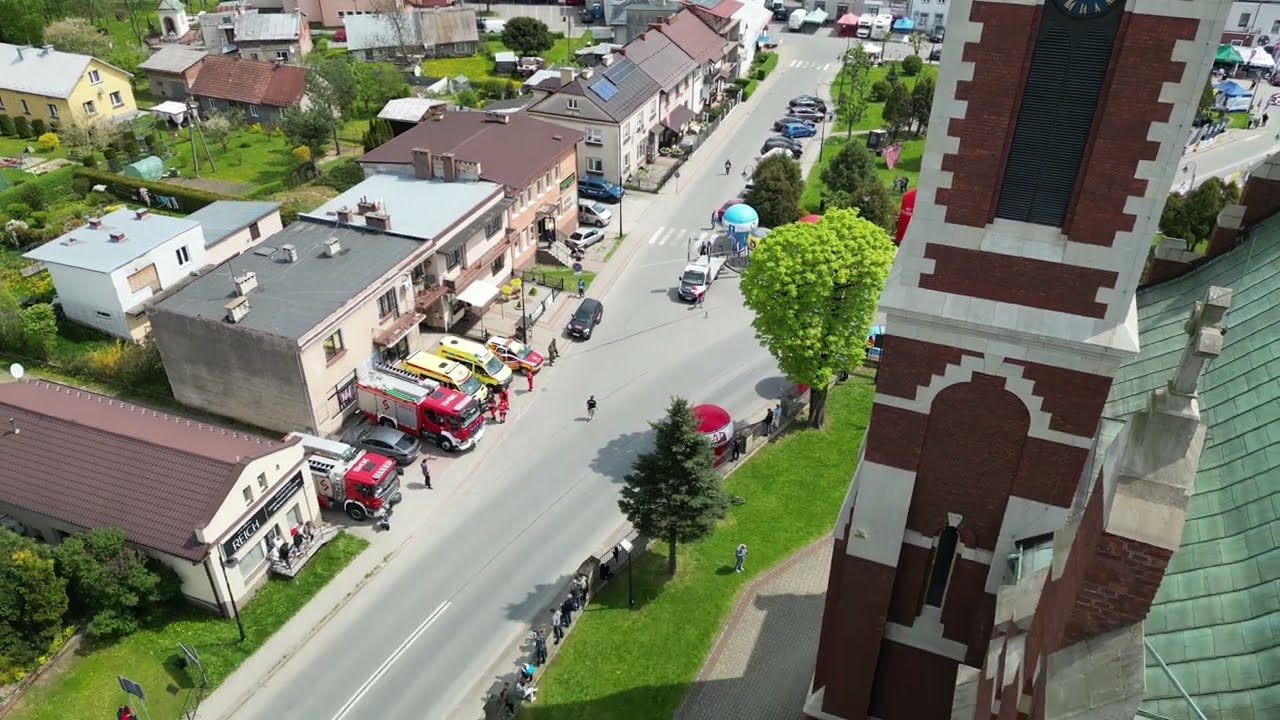This overhead image captures a vibrant portion of a city or small town, bustling with activity on a clear summer day. Dominating the foreground is a striking church steeple, constructed of red and white brick, topped with a green, possibly copper, roof, and adorned with a concrete cross. The steeple also features the edge of a clock face. Surrounding the church is a well-manicured green space, dotted with trees casting long shadows across the grass and road.

Adjacent to this green area is a road that curves gently to the right before continuing straight, lined with a variety of buildings. On the lower left corner of the image, a building prominently displays the word "REICH." Across the street, there is significant activity around what seems to be a fire station, evidenced by the presence of red and white fire trucks and two yellow Sprinter van ambulances. The scene is teeming with life as numerous people walk along the sidewalks and even in the street, weaving between the multitude of parked cars of various colors including blue, black, white, and gray. 

In the background, more buildings stretch out, their rooftops ranging in shades from gray to red and brown. Notable among them is a distinctive blue water tower standing at street level. This highly detailed image captures the essence of a lively residential neighborhood enveloped in greenery and bathed in the warmth of the sun.